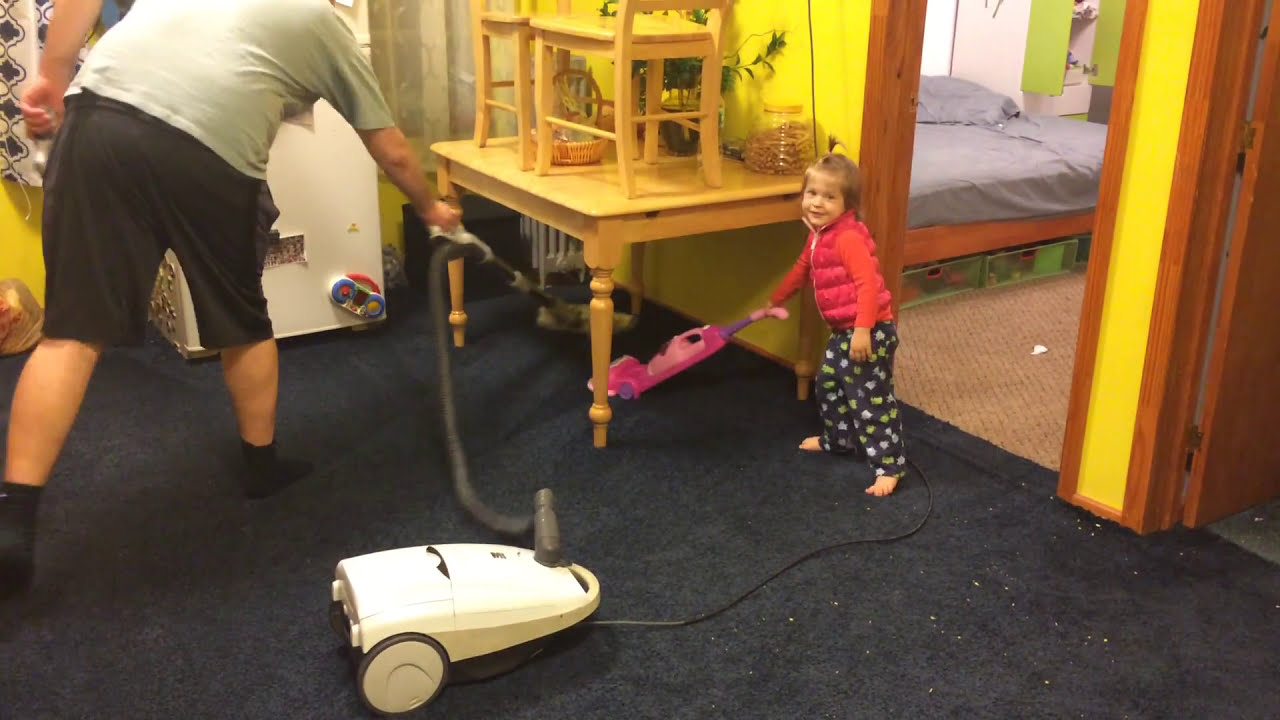In this image, a Caucasian man wearing a gray t-shirt, black shorts, and black socks is using a white and gray vacuum cleaner to clean a blue-gray carpet under a table. The table has chairs placed upside down on top of it, along with a plant and a basket. A small girl, dressed in a pink vest, orange top, and gray pants with patterns, is smiling and using a pink and purple toy vacuum to help the man. The room has yellow walls, wood trim on the doors, and a small refrigerator on the left side with a magnetic child's toy on it. Above the man's arm, there's a curtain, and in the background, there's an open doorway revealing a bedroom with a platform bed covered in gray bedding, green drawers underneath, green cabinets, and white walls or closet doors. To the far right, another doorway is visible, adding depth to the cozy, lived-in scene.